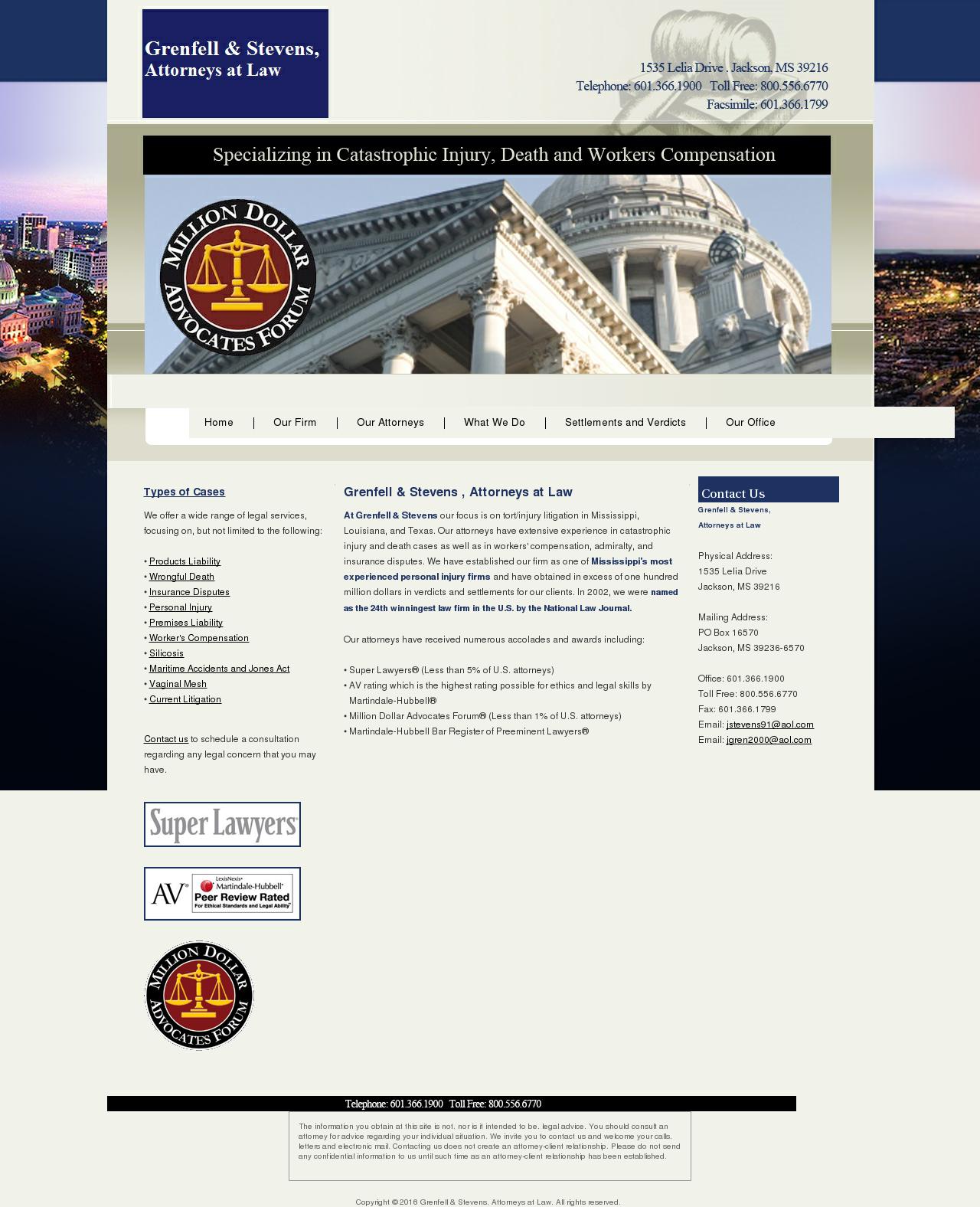The image displays a web page with a prominent central banner at the top. The background of the page is a beige color. At the center of the page, there's a blue square with the text "Grenfell and Stevens Attorneys at Law." To the right, there is an image of a gavel along with the address, phone number, and fax number of the law firm. 

Flanking the sides of the page are banners that extend downward, showcasing a cityscape with clear skies and buildings. Below the top banner, there is a black horizontal banner with white text that reads, "Specializing in Catastrophic Injury, Death, and Workers' Compensation." 

Embedded within this banner is a round black circle with white print that says "Million Dollar Advocates Forum," featuring a red emblem with scales symbolizing the justice system.

Below the banners and central content areas, there's a navigation menu with links labeled "Home," "Our Firm," "Our Attorneys," "Settlements and Verdicts," and "Our Office." Further down, the page details the types of cases the firm handles and provides the full mailing address, phone numbers, and additional contact information for "Grenfell and Stevens Attorneys at Law."